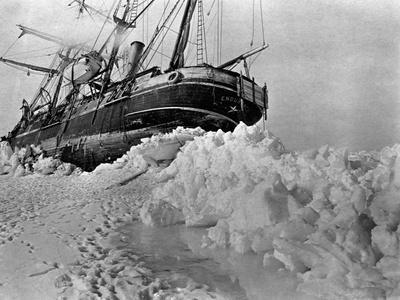This black and white photograph depicts an early industrial steamship with both sail masts and a single smokestack, appearing stranded in a frozen, icy expanse, likely in the Arctic region. The ship, constructed partially of wood and possibly metal, is topped with rolled-up sails, and numerous ropes are visibly leading up and attaching to the masts. The dark-hued vessel is highlighted by a white stripe around its top. The surrounding environment emphasizes the stark conditions: dense, snow-covered ice builds up around the ship's hull, suggesting it’s partially tilted due to the encroaching ice. In the foreground, snow is piled up with small footprints dotting the surface, possibly left by animals or crew members. Men are seen standing on the thick ice around the vessel. The vintage nature of the image is enhanced by the steam visibly emitting from the smokestack, indicating the ship's steam engine is still active despite its predicament. The desolate backdrop and absence of visible water emphasize the isolation and harshness of the scene.